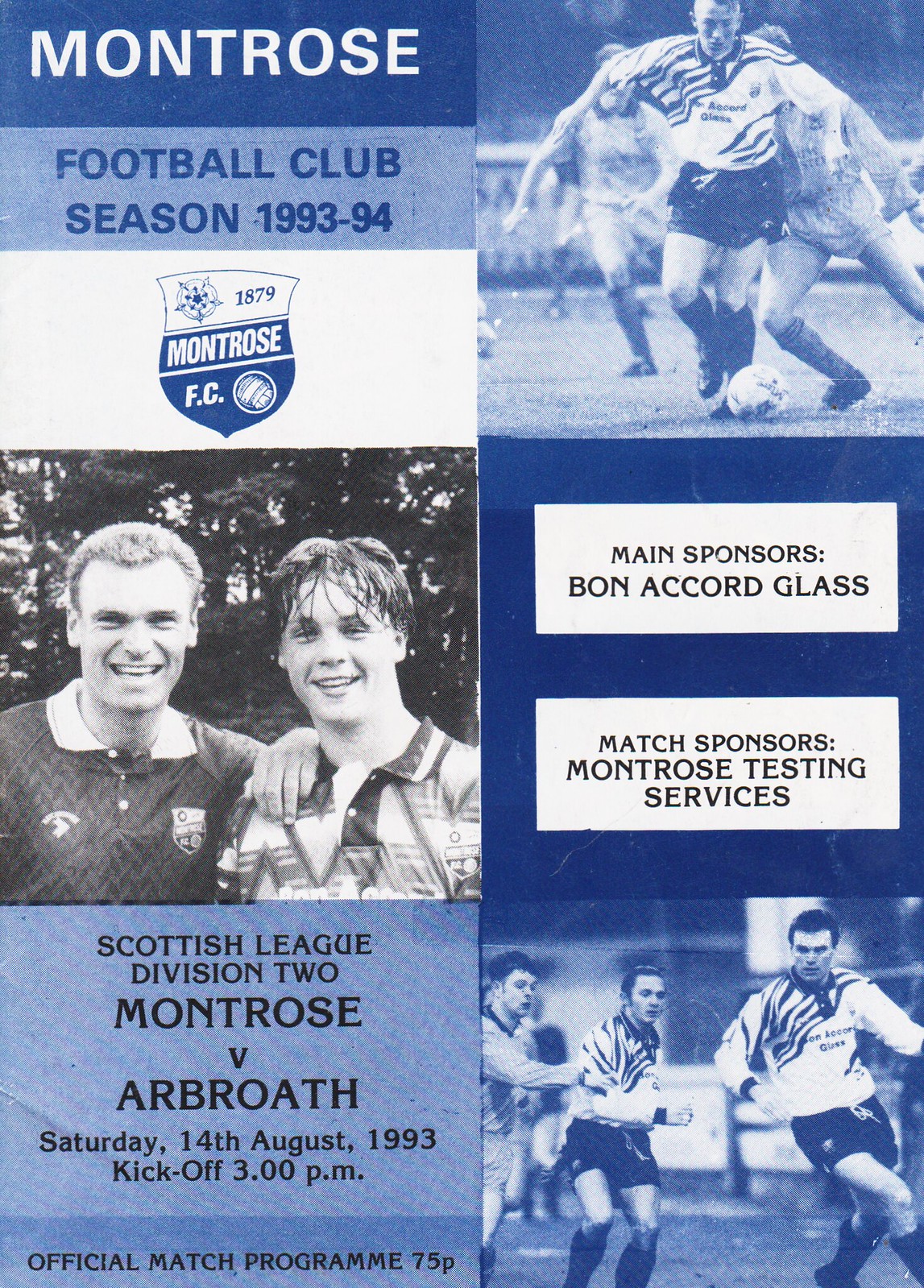This image is an advertisement for the Montrose Football Club's 1993-94 season, presented in a collage style with a mix of light blue, sky blue, black, and white backgrounds. The flyer is segmented into six evenly spaced squares. In the top left square, light blue in color, white text reads "Montrose Football Club Season 1993-94," alongside the club's crest featuring "1879 Montrose FC." To its right, a monochrome sky blue photo depicts three footballers, with one kicking a soccer ball. The center square, in black and white, shows two smiling football players posing together, one with his hand on the other's shoulder, against a background of bushes or trees. To the right, text reads "Main Sponsors Bon Accord Glass" and "Match Sponsors Montrose Testing Services." In the bottom left square, a blue background with black text states "Scottish League Division II Montrose vs. Arbroath, Saturday 14th August 1993, Kickoff 3 p.m. Official Match Program 75 pence." Finally, the bottom right square, sky blue in color, features a photo of three footballers on a field with a distant building in the background, with one player running while the other two chase after him. The poster uses visual and textual elements effectively to promote the football club and its upcoming matches.